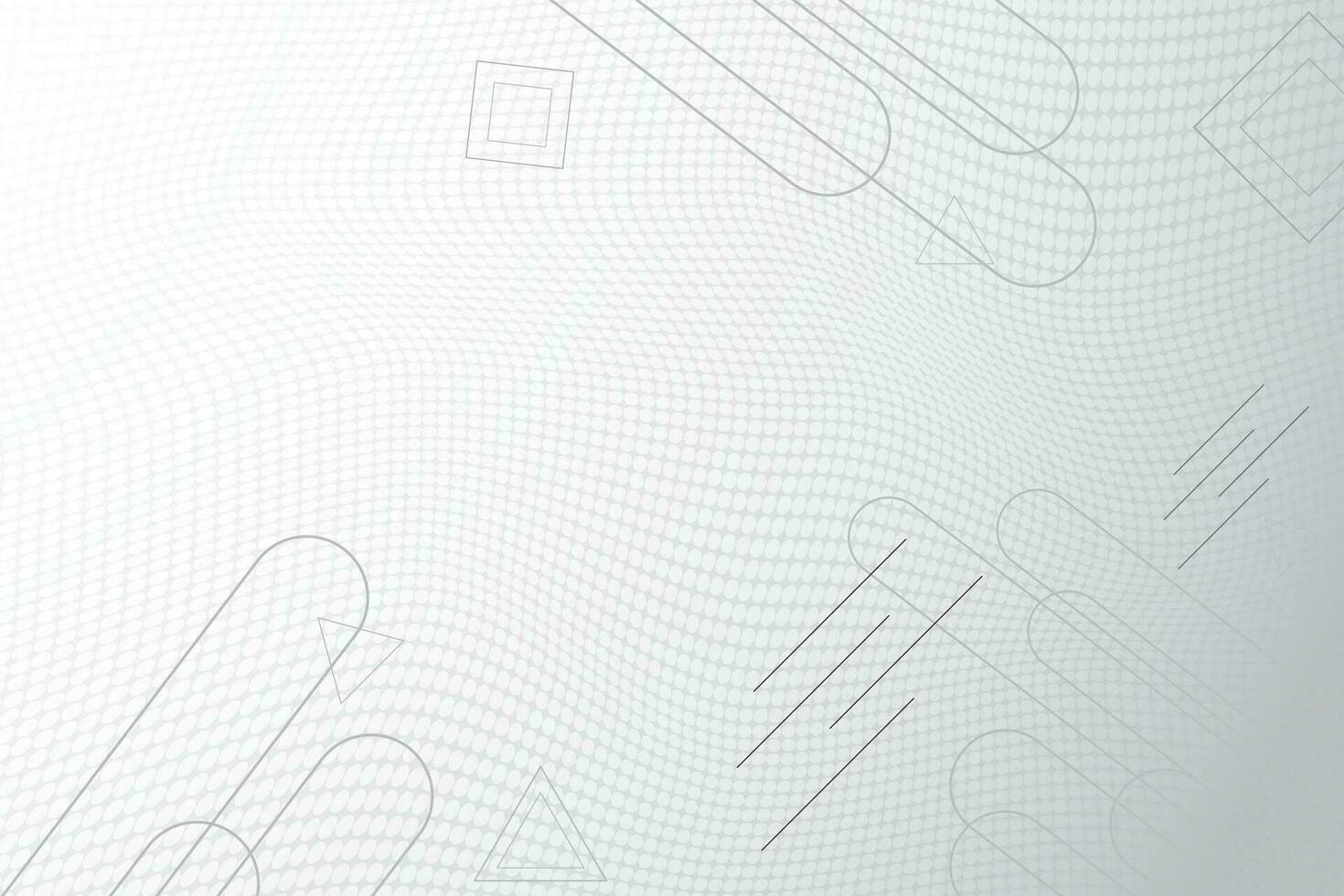The image is a grayscale digital artwork with an abstract, geometric design. The background features a wavy, undulating grid pattern that creates a 3D effect. Across the surface of the image, small white dots form swirling patterns, with lines of dots changing direction to indicate movement. Various geometric shapes overlay the background: there are multiple shapes resembling elongated ovals or tongue depressors, primarily emerging from the bottom left, bottom right, and top center of the image, all pointing towards the middle. These shapes are accompanied by a variety of outlined squares, some nested within each other like picture frames, and triangles, including 3D triangular forms. The lines and shapes are very light gray to black, adding to the delicate yet intricate composition of the artwork. Overall, the arrangement of the shapes and lines is aesthetically pleasing and gives the impression of a meticulous, abstract diagram or design, possibly suitable as a computer background.